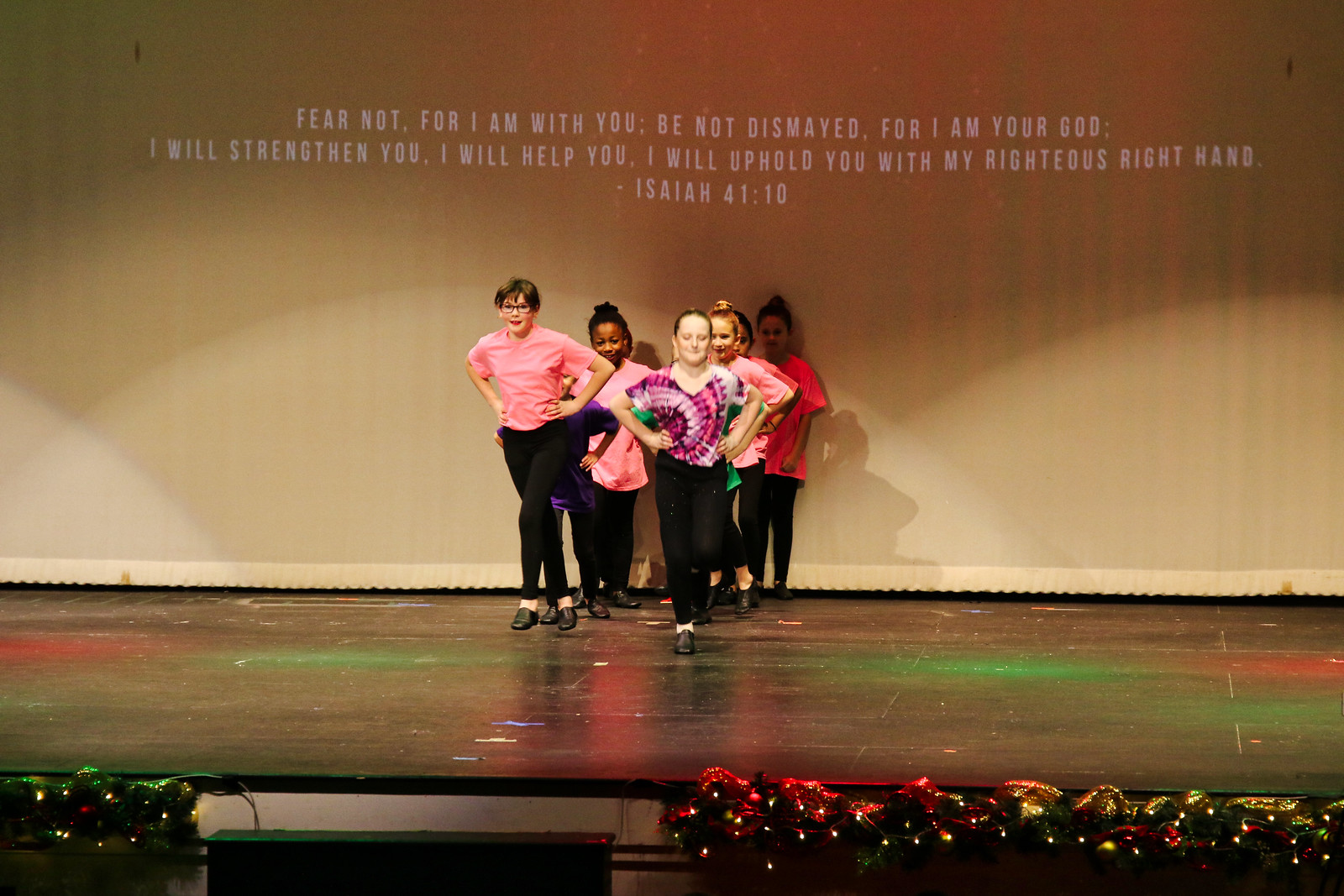Six children are standing on a black stage, lined up in two rows and wearing bright colored tops and black pants. Some of them are dressed in shades of pink, purple, and green, with one girl on the front right in a pink and purple tie-dye shirt and black tap shoes. Behind them, a projector screen displays the text in all caps: "FEAR NOT, for I am with you. Be not dismayed, for I am your God. I will strengthen you, I will help you, I will uphold you with my righteous right hand. Isaiah 41:10." The stage is adorned with bright, shiny items in red, gold, and green at the base, illuminated by various stage lights on the bottom left and right corners, suggesting the scene is part of a performance.